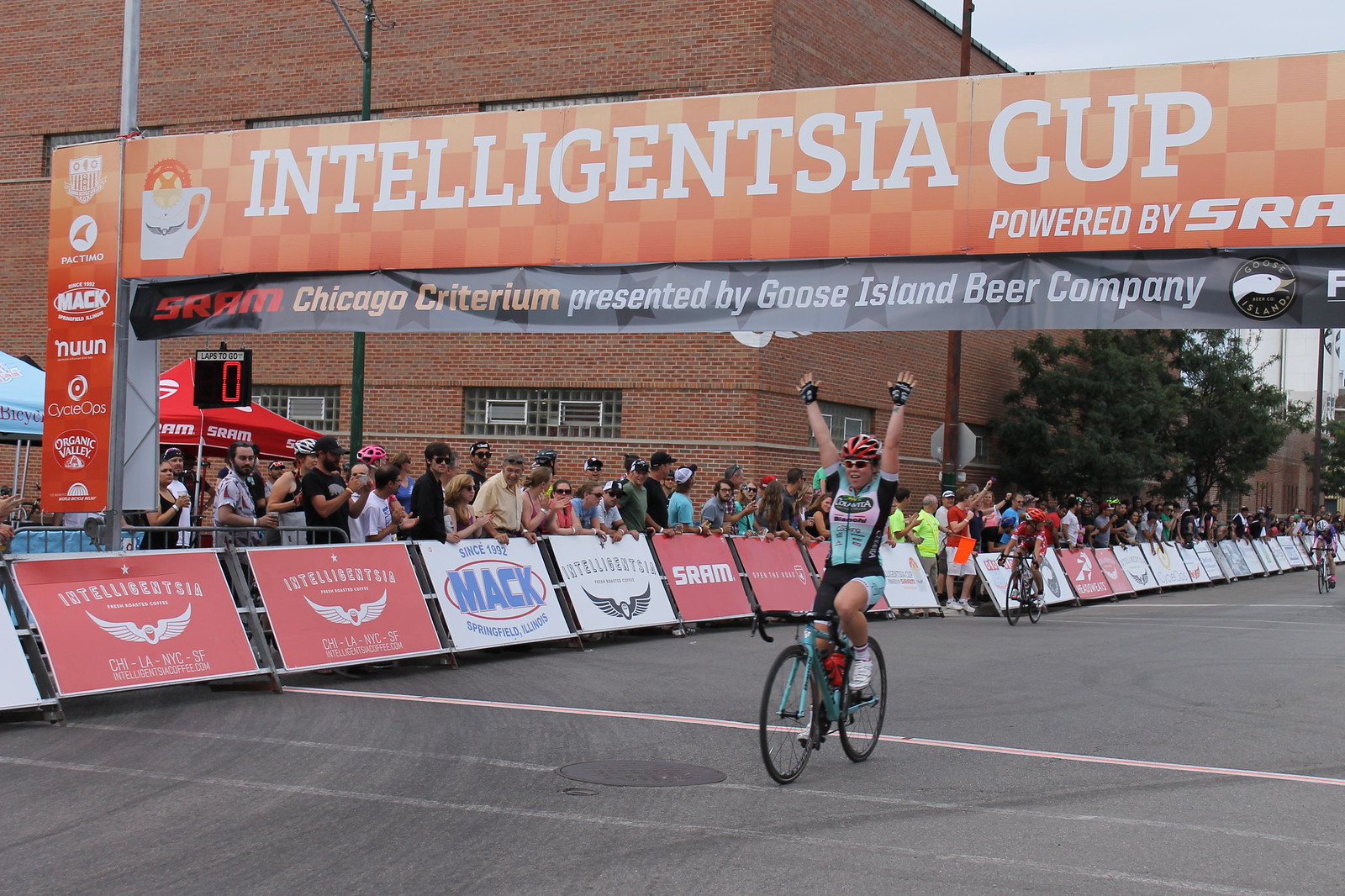This photo captures the exhilarating moment a female cyclist crosses the finish line at the Intelligentsia Cup, specifically the SRAM Chicago Criterium presented by Goose Island Beer Company. Riding a teal bicycle, she celebrates her triumph with arms raised high. She is outfitted in black and white gloves, a red, white, and black helmet, red, black, and white glasses, and a striking pink, teal, black and white spandex ensemble. Her white tennis shoes add a final touch to her vibrant gear.

The finish line is demarcated by an orange banner above, inscribed with "Intelligentsia Cup," followed by details of the event’s sponsors: SRAM and Goose Island Beer Company. The banner has additional writing in black and red on a varied background.

Flanking the race route are barricades adorned with multi-colored advertisements, primarily with red and white backgrounds. Spectators cheer behind these barriers, contributing to the electrifying atmosphere. They consist of fans sporting variously colored t-shirts and bike helmets, watching intently. A backdrop of canopy tents, a brick building with glass-blocked windows, and a couple of trees under an overcast sky frame the jubilant scene. In the distance, two other cyclists with white and red helmets are seen approaching the finish line on the cement street, adding to the race’s dynamic energy.